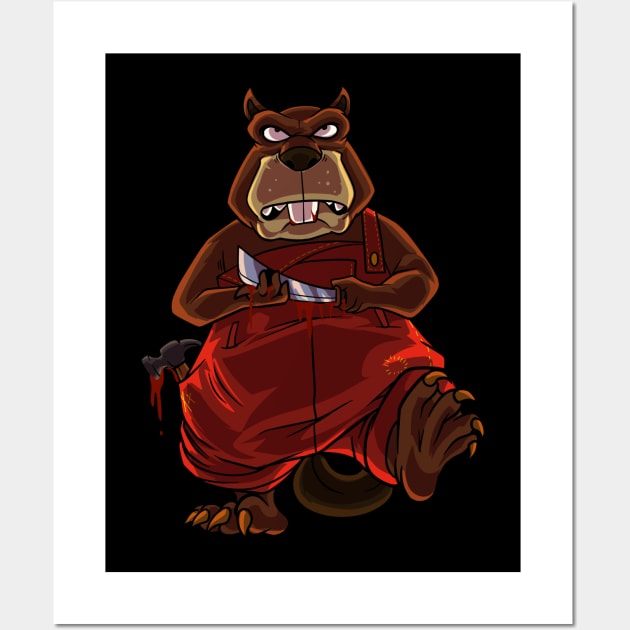In a dark, ominous setting featuring a black background bordered by white and framed with gray rectangular sides, stands an anthropomorphized mammal, possibly resembling a groundhog or a bear-like dog. This menacing creature, predominantly brown with dark and light brown highlights, exudes a sense of hostility with its angry, narrowed eyes and exposed sharp canines adjacent to its prominent buck teeth. It is clad in red overalls, secured by a single brass button strap while the other dangles loosely. From its left overall pocket protrudes a claw hammer, its head smeared with a red, blood-like substance. Gripped firmly in both of its clawed hands is a squared-blade cleaver, also dripping with fresh blood. The creature is shown standing on its hind legs, revealing four sharp claws on each foot and a long bushy tail extending between them, heightening the sense of dread and danger in this detailed cartoon-style depiction.